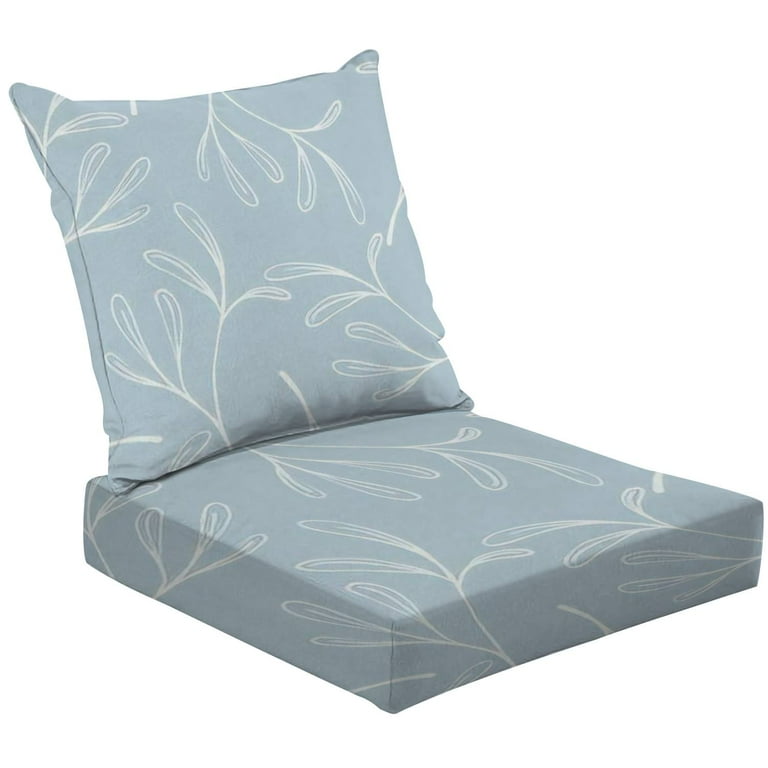The image features a professional promotional photo of a portable seating arrangement that includes a cushion and a backrest pillow. Both the cushion and the backrest are square-shaped and exhibit a soft green color with a delicate pattern of white plant silhouettes, featuring long, swaying leaves. The photo is set against a plain white background, emphasizing the design and color of the seating pieces. The heavily padded cushion forms a comfortable seat, while the less cushioned backrest pillow is positioned diagonally, leaning towards the left as if against an unseen wall to simulate support. This seating arrangement appears designed for floor use, providing a compact and stylish solution for lounging, possibly while watching television.